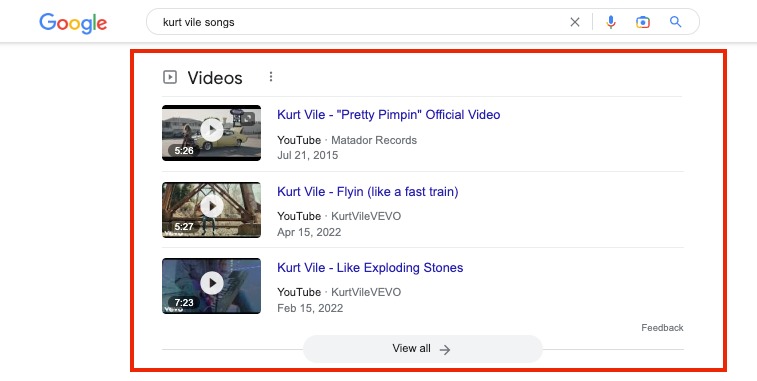This image is a screenshot from the Google website. In the top-left corner, the Google logo is prominently displayed with the iconic color scheme: a blue "G," a red first "O," a yellow second "O," a blue "G," a green "L," and a red "E." To the right of the logo is the search bar containing the query "Kurt Vile songs," spelled out as "K U R T V I L E." Adjacent to the search query are an "X" icon, a vertical line, a microphone icon, a camera icon, and a magnifying glass icon.

The background of the page is white. Below the search bar, a red rectangular border highlights the search results section. At the top of this section is a toolbar featuring a square icon, a right-facing triangle labeled "Videos," and a set of three vertical dots.

The search results list three video entries:
1. **Kurt Vile - Pretty Pimpin (Official Video)**
   - Platform: YouTube
   - Channel: Matador Records
   - Date: July 21, 2015
   - View Count: 526K

2. **Kurt Vile - Flyin (like a fast train)**
   - Platform: YouTube
   - Channel: Kurt Vile VEVO
   - Date: April 15, 2022
   - View Count: 527K

3. **Kurt Vile - Like Exploding Stones**
   - Platform: YouTube
   - Channel: Kurt Vile VEVO
   - Date: February 15, 2022
   - View Count: 723K

Beneath the video results, there is a banner with the text "View All" and an arrow pointing to the right, indicating additional results can be accessed.